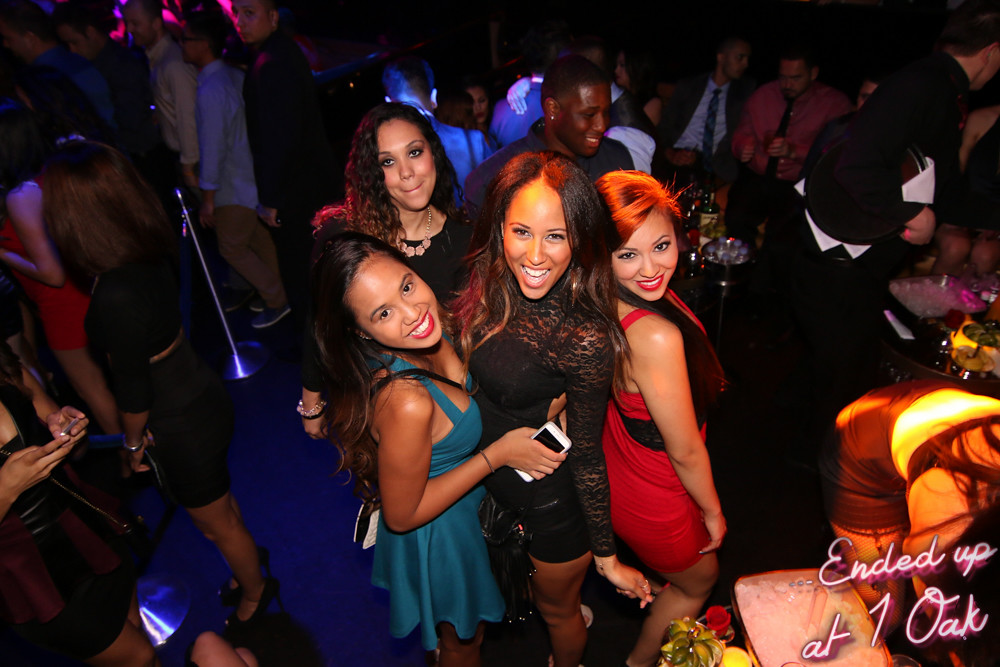In this vibrant photo taken at a bustling nightclub, a central group of four young women pose together, drawing immediate attention. The women are warmed by cheerful smiles and dressed to impress. At the center stands an African American woman with dark hair, wearing a black lace top and matching shorts, grinning up at the camera. To her left is a shorter woman with dark hair in a striking blue dress, holding a phone in her right hand and looking up with a bright smile. On her right is an Asian woman with striking red hair, donned in a matching red dress, back-to-back with her friends. Behind them, slightly to the left, is a woman with curly brown hair, wearing a black dress and a necklace, tilting her head and grinning subtly. The nightclub's blue floor underlines the lively atmosphere, with numerous other guests scattered in the background, some standing, some seated, many holding phones or drinks. A table nearby is laden with various alcoholic beverages, adding to the festivity. The scene is illuminated by a text at the bottom right in neon-like lettering that reads, "Ended up at One Oak."